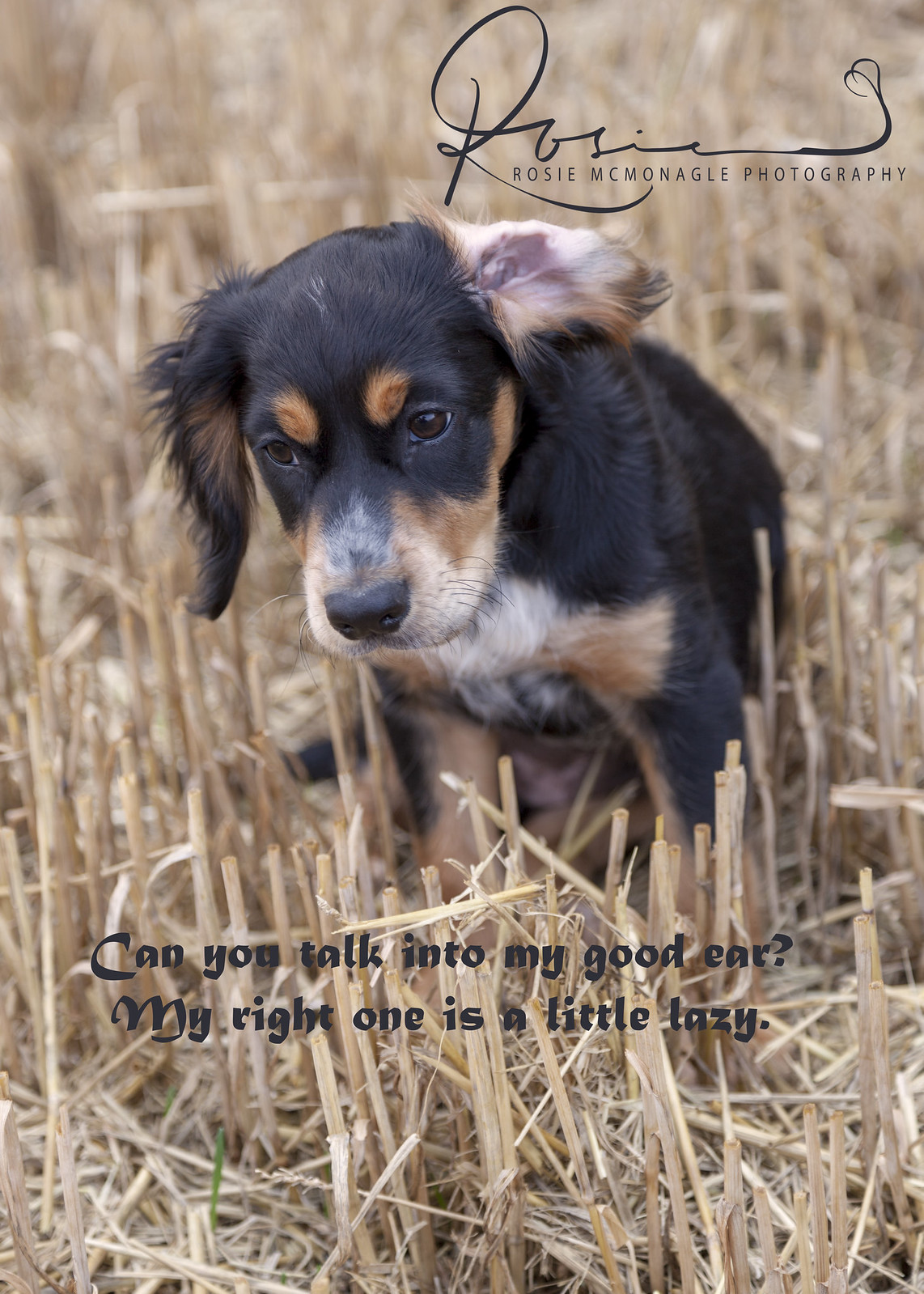This image features an adorable black and tan spaniel puppy with a touch of white on its chest and muzzle. The puppy sits quizzically in a field of straw-like, cut reeds or wheat, with its left ear comically bent back, exposing the inside of the ear canal, while its right ear hangs down normally. The puppy's expressive face seems to reflect the caption below the image, which reads in black text, "Can you talk into my good ear? My right one is a little lazy." In the upper right-hand corner, the photographer's signature is elegantly scripted, most likely reading Rosie McConagall Photography, though its exact legibility is uncertain. The image, rectangular and slender in shape, could be a scan of a greeting card, a screen grab from a website, or a handout for the photographer's business.